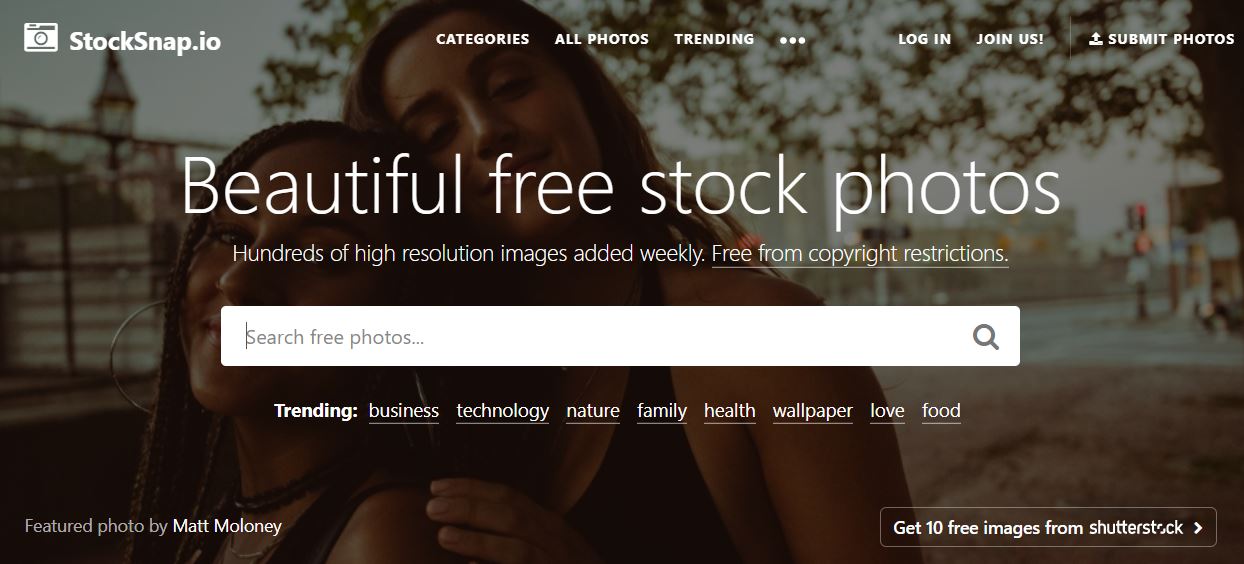The main page of a stock photo website, StockSnap.io, is presented with a stylish and modern interface. The background of the page features a dark, slightly saturated photo of two women embracing in what appears to be a city park at night. One woman stands in front of the other, both leaning into each other, creating a warm, intimate scene.

In the upper left corner, the StockSnap.io logo and icon are displayed prominently. To the right, there are various navigation options including categories, a login button, a "Join Us" link, and a "Submit Photos" button.

Centrally over the background image, in elegant thin white text, the main headline reads: "Beautiful free stock photos." Following this, it states: "Hundreds of high-resolution images added weekly, free from copyright restrictions."

Beneath this headline is a white search bar labeled "Search free photos" accompanied by a search icon. Below the search bar are trending topics listed in white text: "Trending, Business, Technology, Nature, Family, Health, Wallpaper, Love, and Food."

In the lower left-hand corner, a caption reads: "Featured photo by Matt Maloney." On the lower right-hand side, enclosed in a white-bordered box with thin white text, there is a call-to-action button that says: "Get 10 free images from Shutterstock," accompanied by an arrow pointing to the right. The overall design is characterized by its clean, modern look, with a stark contrast between the dark background and the white text.